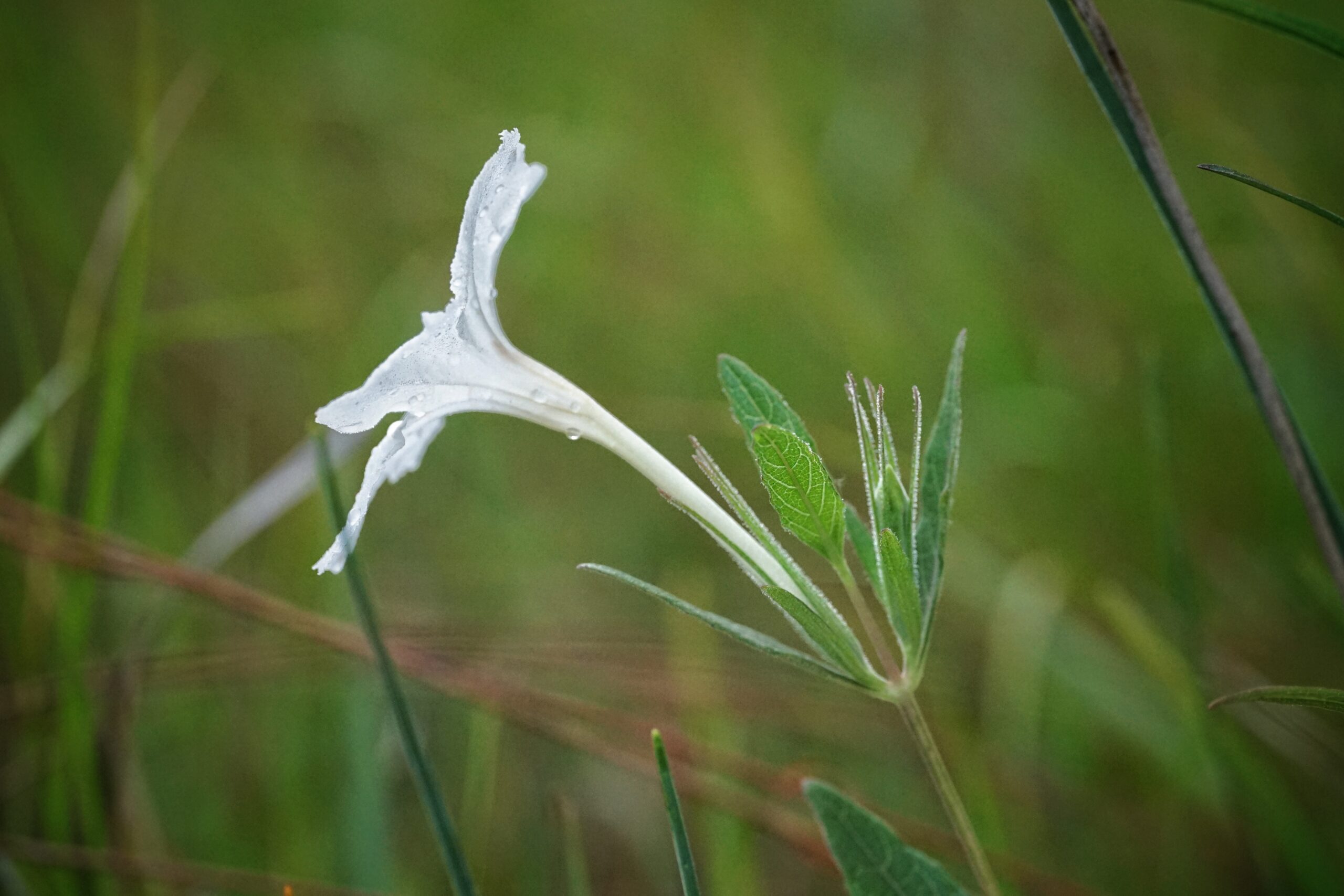This professionally taken photograph captures a serene outdoor scene in natural daylight, likely on an overcast day due to the soft lighting. The composition is horizontally rectangular with no border, focusing on a white flower emerging amid a blurred, lush green background of various plants and tall grasses. The background features a mix of green and brown vegetation, contributing to the image's natural setting.

In the upper right corner, a brown stalk or stem descends diagonally to just below the middle of the photo. The lower right corner has a thin green leaf peeking out. Near the bottom, left of the thin leaf, a green stalk with pointed leaves appears, forming a ring around the centerpiece of the image—a delicate white flower. 

The flower, which could be a small tulip, blooms prominently in the center, standing out against the backdrop due to its bright white, slightly tubular petals that fan out gracefully. The flower's stem is long and green, complementing the various other shades of green from the surrounding leaves. Notably, the flower petals glisten with droplets of dew, suggesting that the photo may have been taken in the morning. The overall depiction is of a tranquil, natural environment with the white flower beautifully contrasted against the verdant background.